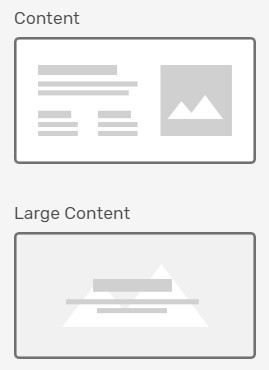The image features an instructional dialog box with a vertically oriented, light gray background. The box is divided into several sections:

1. At the top left, the word "Content" is displayed in a dark gray font.
2. Directly beneath this label is a dark gray rectangle containing a very light-colored (possibly white or off-white) area. This area appears to be the outline of text.
3. To the right of this section is a square icon depicting a gray mountain with a lighter, almost white, mountain in the center, representing an image placeholder.
4. Below this, on the left side, are multiple gray rectangles symbolizing lines of text. 
    - The first line is thicker and aligns horizontally with the top of the mountain icon on the right.
    - Underneath, there is a longer, thinner gray line.
    - Following this, a slightly shorter gray line is present.
5. Further down, there are two columns of gray boxes:
    - The top row has a thicker box on the left and a matching right box.
    - Beneath these, there are two thinner boxes in each column, side by side.
6. At the bottom of the dialog box, the phrase "Large Content" is present.
7. Below this phrase is another rectangle matching the dark gray color used elsewhere in the box. Inside this, there is another mountain icon with gray and white tones similar to the top one, symbolizing another image placeholder.
8. Above this bottom image placeholder, there are three gray rectangles that likely represent text:
    - The first is thicker.
    - The second is longer and thinner.
    - The third is shorter and thin, forming a structured layout within the box.

The dialog box appears to be an organized template for displaying content, imagery, and text on a website.